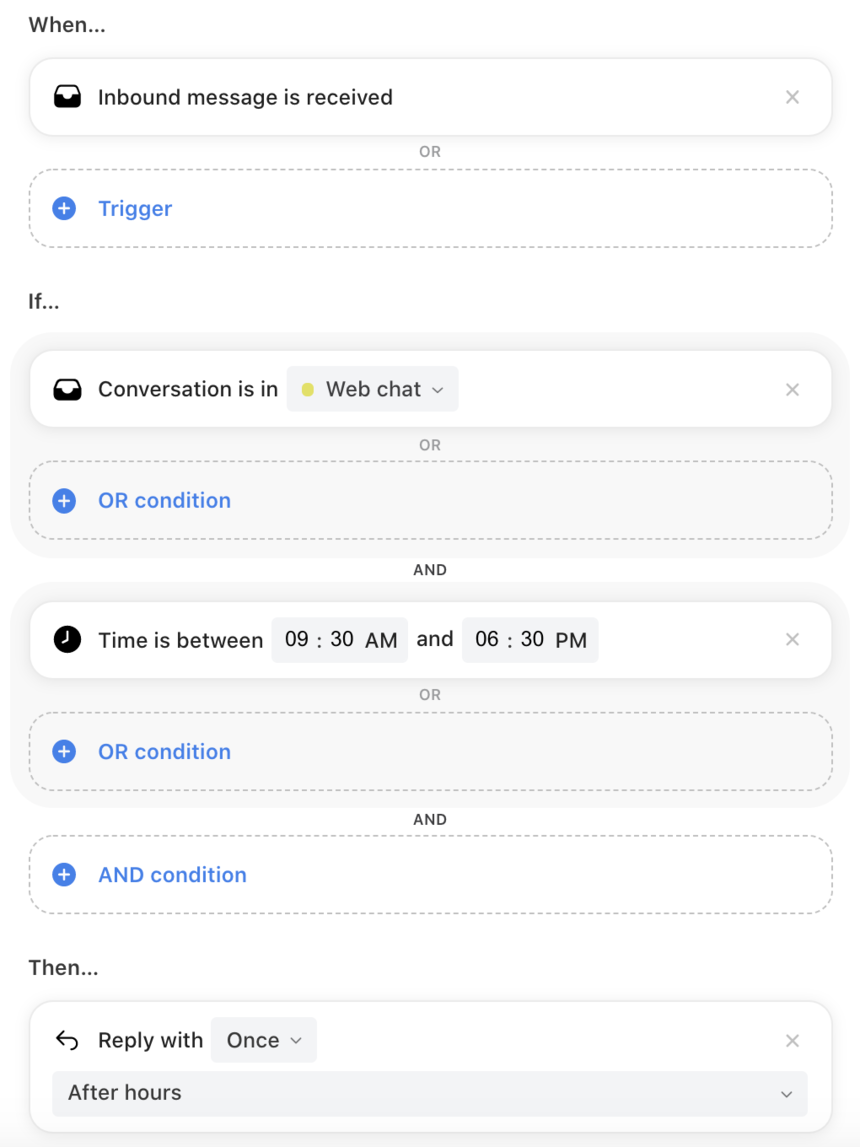This image is a detailed screenshot of a coding sequence, specifically in portrait mode. The interface appears to be part of an automation or chatbot scripting platform.

In the upper left-hand corner, there is a label titled "when." Directly next to it, the tab reads "inbound message is received." Below, the word "or" is displayed in light gray against a white background, making it difficult to read. A blue button labeled "trigger" with a plus sign allows adding another trigger condition.

The sequence continues with, "if conversation is in," followed by a dropdown menu set to "web chat." Again, "or" is displayed in very light grey with an option to "add an or condition" in blue text.

Further down, there's a condition specifying, "time is between 9:30 a.m. and 6:30 p.m." This is followed by another light gray "or," indicating the possibility to add another condition. An "and" condition can also be added via a blue button.

Next in the sequence, there's a back arrow and the text "reply with" followed by a dropdown menu. Underneath, there's an option labeled "after hours" with another dropdown menu.

In summary, the program flow described is:
- When an inbound message is received,
- If the conversation is in web chat and the time is between 9:30 a.m. and 6:30 p.m.,
- Then reply with the predefined "after hours" message.

The described sequence demonstrates the conditional logic and response setup in the script, although it might require additional configuration to function properly.